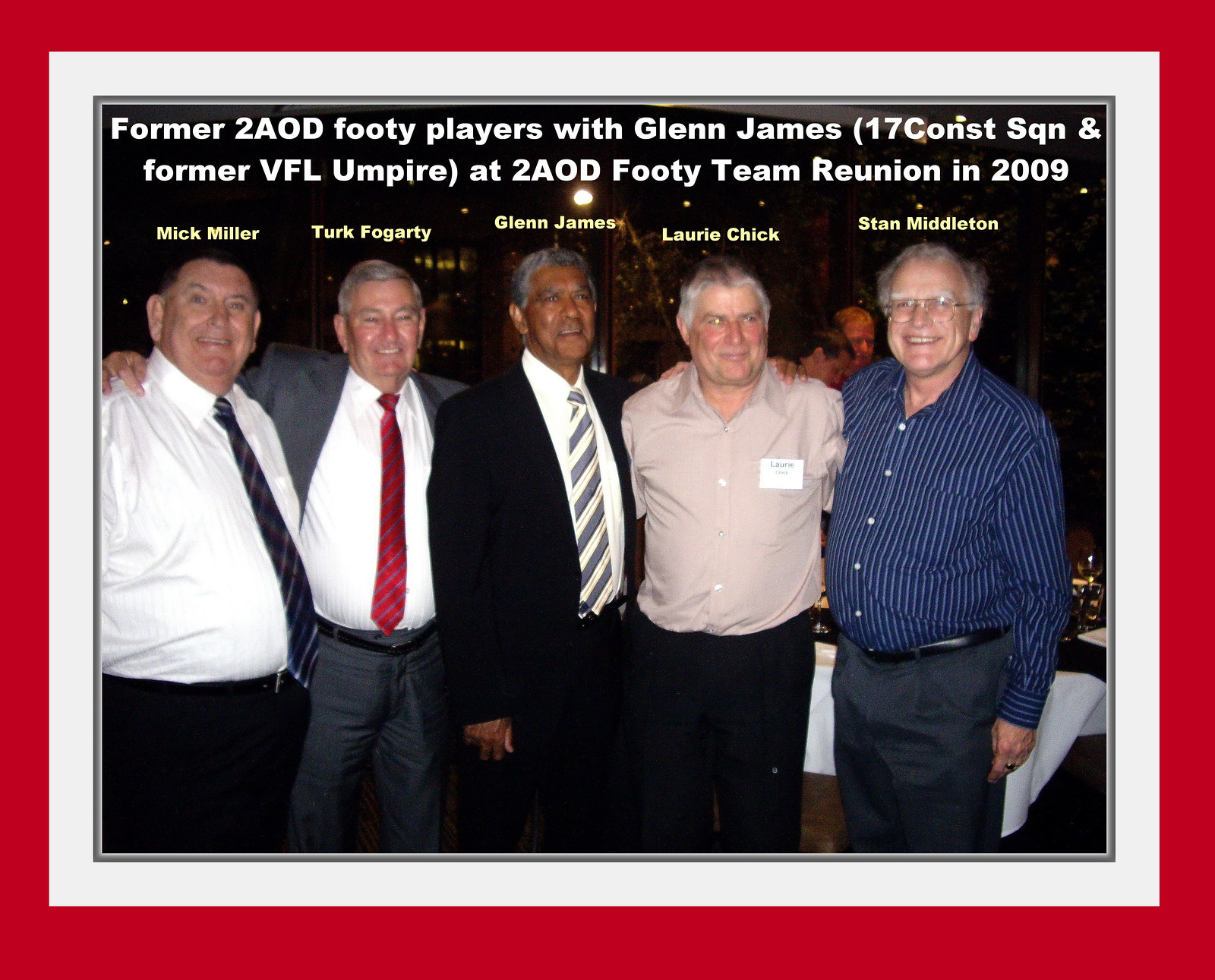This color photograph, set within a layered red, white, and thin gray border, captures a reunion of former Two AOD footy players and Glenn James, a past VFL umpire. The photo, taken in 2009, features five older gentlemen with gray hair, standing side-by-side with their arms around each other, all smiling warmly at the camera. The men are framed against a dark background, which suggests they are indoors. 

At the top, a white headline reads: "Former Two AOD Footy Players with Glenn James (17 CONST SQN) and Former VFL Umpire at Two AOD Footy Team Reunion in 2009." Below this, their names are written in yellow from left to right:
- MacMiller: He is dressed in a white shirt with a dark diagonal striped tie and black pants.
- Turk Foggery: He wears a white shirt, a red tie with darker diagonal stripes, a gray suit coat, and gray pants.
- Glenn James: Distinguished by his darker complexion and gray hair, he wears a dark suit coat and pants, a white shirt, and a tie with gray and cream-colored diagonal stripes.
- Lori Chick: Wearing black pants and a tan-colored shirt, which has a possible name tag on the left pocket.
- Stan Middleton: Dressed in a blue and white vertically striped shirt, dark gray or bluish pants with a belt, and glasses.

This photo utilizes a representational realism style, combining photographic detail with superimposed text to commemorate the moment.